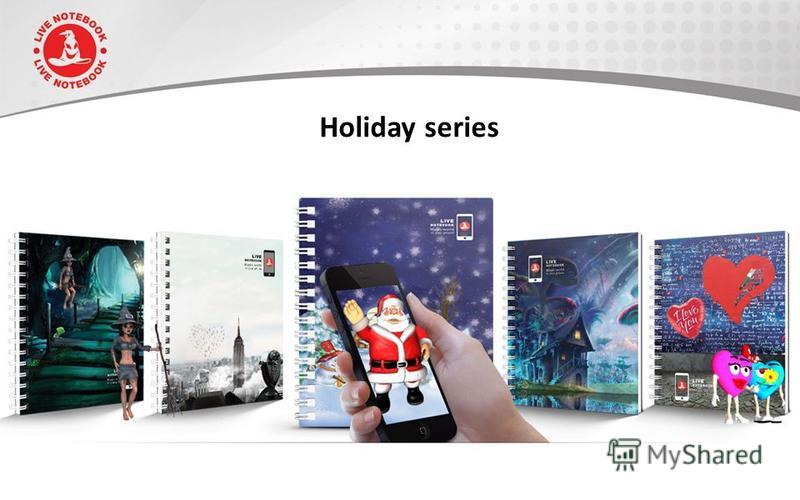The image features a central focus on the text "Holiday Series" in black, positioned slightly above the middle. In the upper left-hand corner, there is a red emblem that reads "Live Notebook" at the top and bottom, encircling an intricate design resembling a witch’s hat with a smiley face. The background fades from a solid gray on the left, streaked into a dotted gray pattern as it moves right. 

Below "Holiday Series," the main background is white, showcasing five books with plastic binders. The first book on the far left has a fairy-tale theme with a character in a gray outfit and hat, holding a brown stick. The next book features a cityscape, followed by a notebook adorned with snowflakes on a blue background. The fourth book displays a majestic magical house, and the fifth has a design with hearts. 

Prominently in the center, a hand holds a smartphone displaying a waving Santa Claus. He is dressed in a red jacket with white fur trim, a white beard, and a red hat. On the bottom right, two heart-shaped cartoon characters add a whimsical touch—one teal and one pink, both with white legs, arms, and eyes.